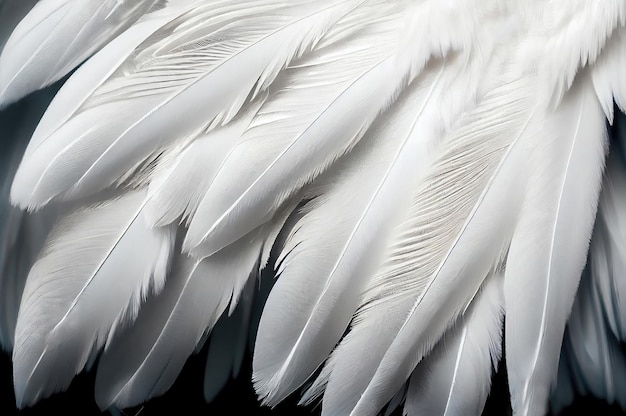The image captures an array of white feathers against a stark, dark background, making the feathers stand out prominently. The close-up shot reveals intricate details, with some feathers appearing soft and delicate, featuring fine fronds, while others are coarser and partially transparent. The lighting highlights a strong central rib in each feather, casting noticeable shadows. The feathers vary in size and texture, creating interesting patterns through layering. Towards the top right corner of the image, there are feathers that look different from the rest, suggesting they might be closer to the bird’s body. This contrast with the more uniform feathers below, which cover the center densely but become sparser towards the bottom, showcases the natural variations within the collection.